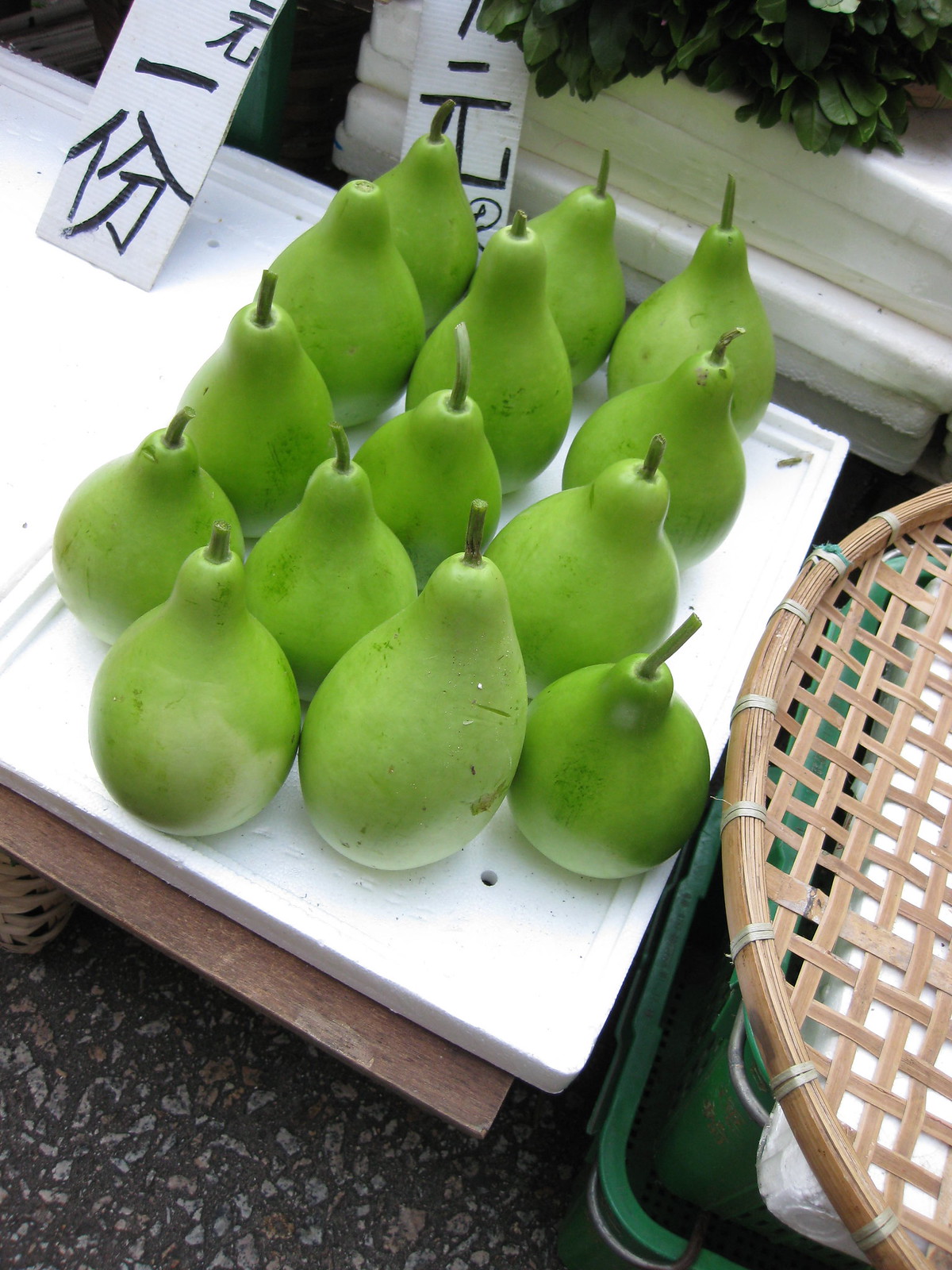This outdoor, daytime color photograph captures a collection of bright green pears neatly arranged on a white serving tray that's placed on a black and gray mottled countertop. The pears are standing upright, organized primarily in rows of three, with an additional row of two, though the rows are not perfectly straight. Each pear has a stem except one in the far top left which lacks it. To the right of the tray, there is the partial view of what appears to be a wicker basket. In the background, on the upper right, white Styrofoam suggests a stack of sheets possibly adorned with green leaves. On the upper left, there are two white tags featuring Chinese characters. The scene, likely at a yard sale, is framed by a green container visible beneath the white tray and subtle hints of gravel or dirt in the lower right corner.